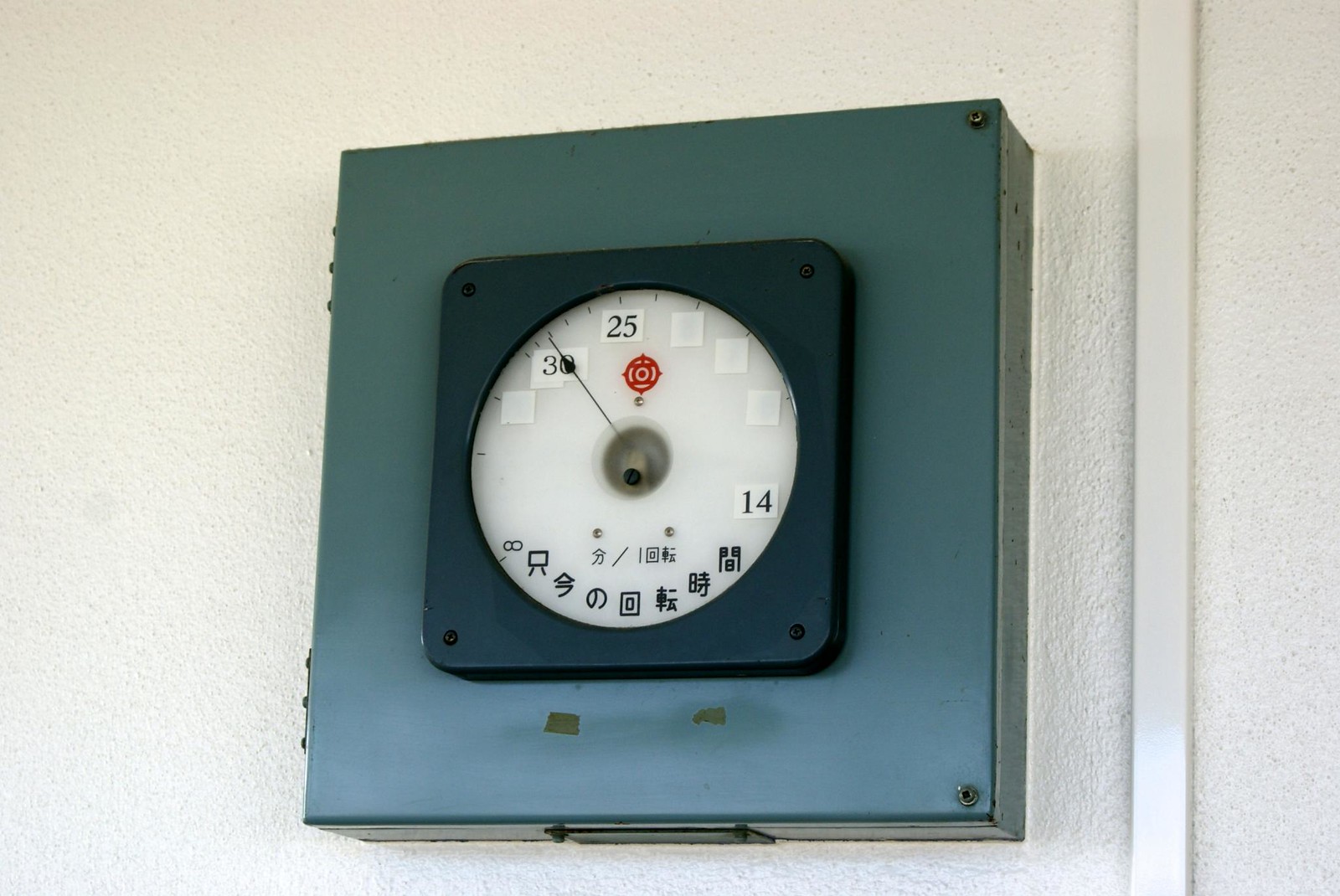This photograph features a large green square metal box attached to a white wall. In the upper right and left-hand corners of the box are visible Phillips head screws. At the center of the green box is a black square with rounded corners, which houses a detailed interface.

In the center of the black square, there is a white circular dial resembling a clock face. At the core of this white circle, a gray disc is visible, from which a small gray cylinder extends outward. This cylinder has a black circle at its tip.

Along the bottom edge of the white circle are various characters. Specifically, at the position where the 4 o'clock mark would normally be located on a traditional clock, there is a black number "14" inside a white square. In the positions corresponding to 1, 2, and 3 o'clock, there are plain white squares. Extending from the gray cylinder in the center of the circle is a single black hand, which appears to be pointing between the number "3" and the next character.

At the top position, where the 12 o'clock mark would normally be, there is a black number "25" within a white square. Below this, where the 10 o'clock position would be, the number "3" is displayed in black. The black hand is positioned across the next character in sequence.